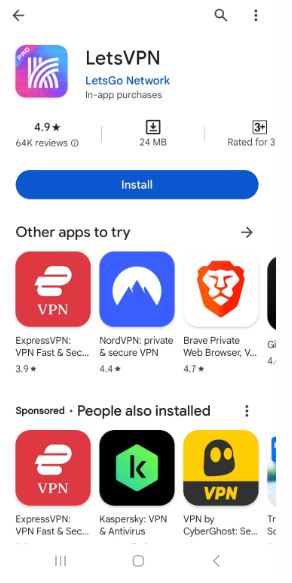The image depicts a smartphone screen displaying a listing for a VPN application in an app store. The application, "Let's VPN," is highlighted prominently. The icon for "Let's VPN" features a purple square with rounded edges, containing three white diagonal stripes that converge to the top right. To the right of the icon, in black text, it reads "Let's VPN," followed by "Network" in blue text. Beneath the name, it notes that there are in-app purchases available.

The app has an impressive rating of 4.9 stars based on 64K reviews. Directly to the right of this information, there is a download button indicating the app's size as 24 megabytes, and it's suitable for users aged 3 and above. Below this button, a blue "Install" button is prominently displayed.

Further down the screen, there are three other suggested applications: ExpressVPN, NordVPN, and the Brave Private Web Browser. These are categorized under "Sponsored" and "People also installed," suggesting that users who downloaded "Let's VPN" also showed interest in these applications. The listing signifies one of the popular VPN applications, "ExpressVPN," as another notable recommendation.